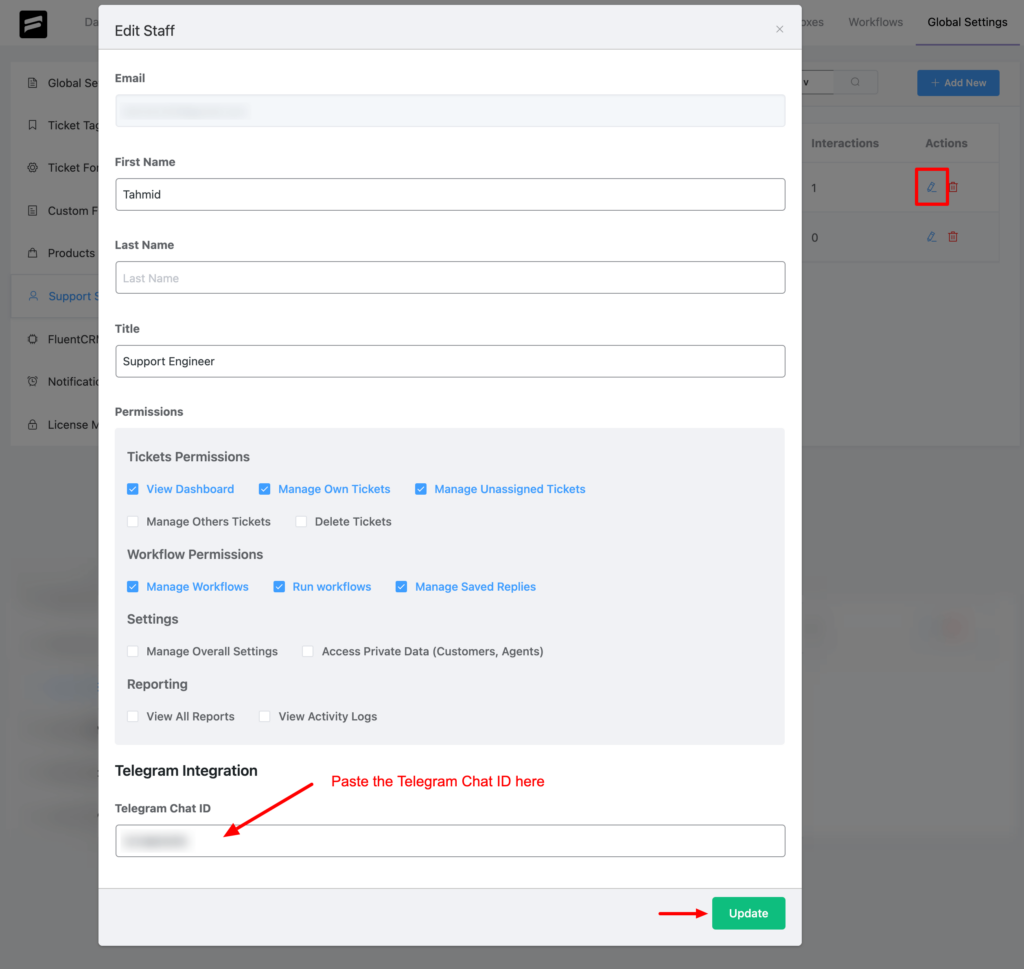Sure, here's a cleaned-up and detailed version of the caption:

"Screenshot of a staff edit interface. The interface has a gray border at the top labeled 'Edit Staff'. Below that, fields for 'Email' and 'First Name' are displayed, with the latter pre-filled with 'Tamid'. The 'Last Name' field is pre-filled with 'last name'. The 'Title' field contains 'Support Engineer'. Further down, a section labeled 'Permissions' contains a list of options including 'View Dashboard', 'Manage Own Tickets', 'Manage Unassigned Tickets', 'Manage Other Tickets', 'Delete Tickets', 'Workflow Permission', 'Manage Workflows', 'Run Workflow', 'Manage Saved Replies', 'Settings', 'Manage Overall Settings', 'Access Private Data', 'Customers', 'Agents', 'Report', 'View All Reports', 'Do Activity Logs', 'Telegram Integration', and 'Telegram Chat ID'. Text boxes for entering specific data are visible, with one for the 'Telegram Chat ID' highlighted by a blurred privacy effect and a red arrow pointing to it with a note to paste the ID. A green 'Update' button is positioned at the bottom, with another red arrow pointing towards it."